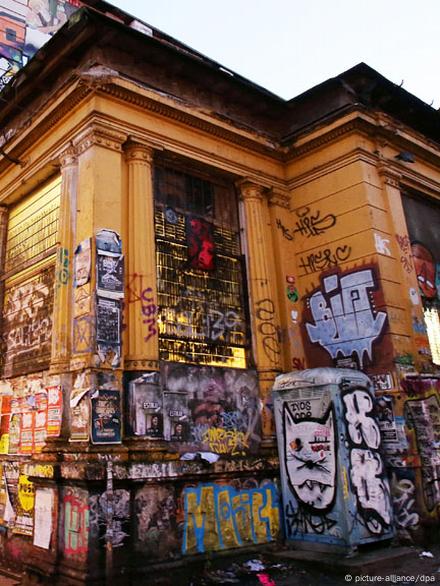This is a photograph of the exterior of a heavily graffitied building taken during the daytime. The building itself is constructed from dark orange bricks and has an unusual structure, with a smaller rectangular section protruding and a wider rectangular section extending beside it. The clear blue sky visible at the top of the vertically-oriented image indicates it is daytime. 

The lower half of the building is covered in a vibrant array of graffiti featuring a variety of colors and designs. Among the graffiti, a prominent white cat face is noticeable, alongside various writings in black, blue, and yellow that are difficult to decipher. Additionally, some red graffiti and squiggly lines are scattered across the wall. 

There are also graffitied pillars and numerous posters attached to the wall, contributing to a distinctly European or UK-like atmosphere. A trash can adjacent to the building also bears some graffiti, including a depiction of a cat. At the bottom right corner of the image, a watermark reading "Alliance DPA" is visible. The chaotic and colorful display of graffiti transforms the building into an urban canvas.